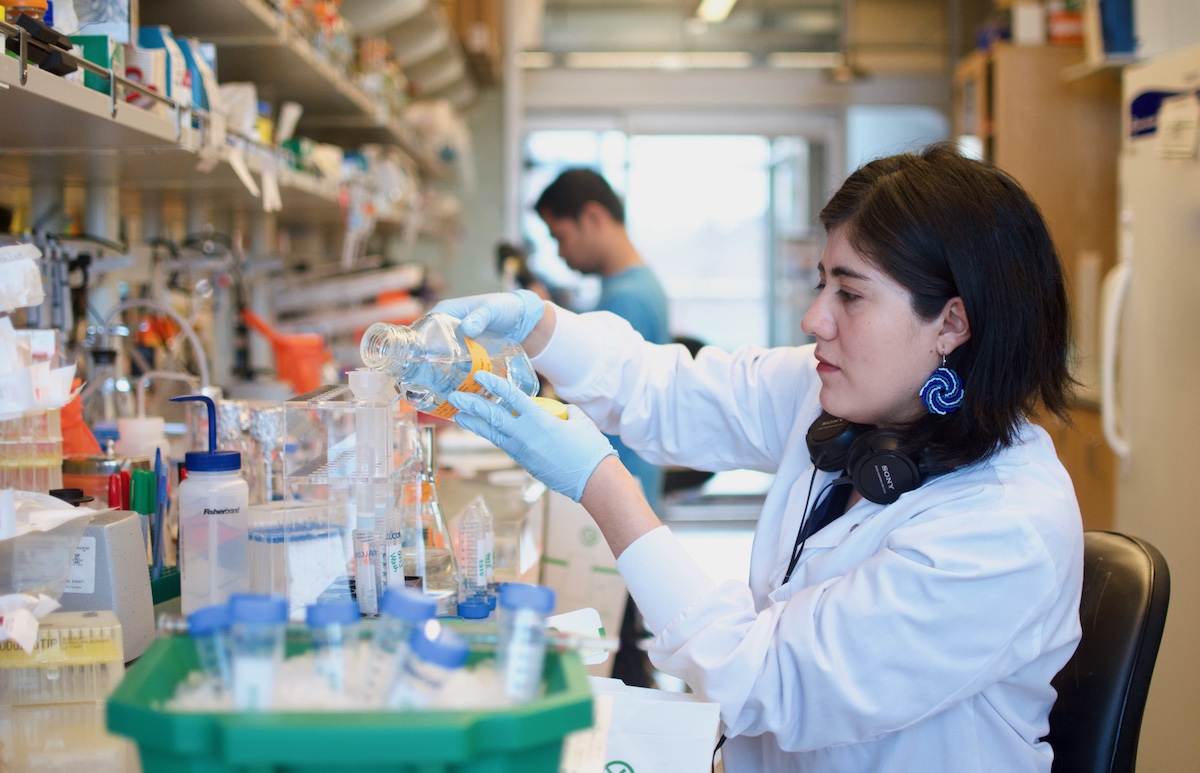In the photograph, a woman is seated in the bottom right corner, working meticulously in a lab setting. She is wearing a white lab coat and has black over-the-ear headphones, with the brand "Bose" visible in white text on the side, resting around her neck. She has striking blue spiral earrings dangling from her ears and short black hair that falls just above her shoulders. Her hands are protected by blue latex gloves as she carefully pours a clear liquid from a square bottle into a funnel that is connected to another bottle in front of her. Arrayed on the table are various tubes, jars, and instruments, with a green tray holding test tubes with blue lids possibly nestled in ice to her left. In the background, blurred but noticeable, another person wearing a blue shirt is also engaged in lab work at the same counter. The setting features ample shelving filled with additional lab equipment, reinforcing the busy, detailed atmosphere of the research environment.